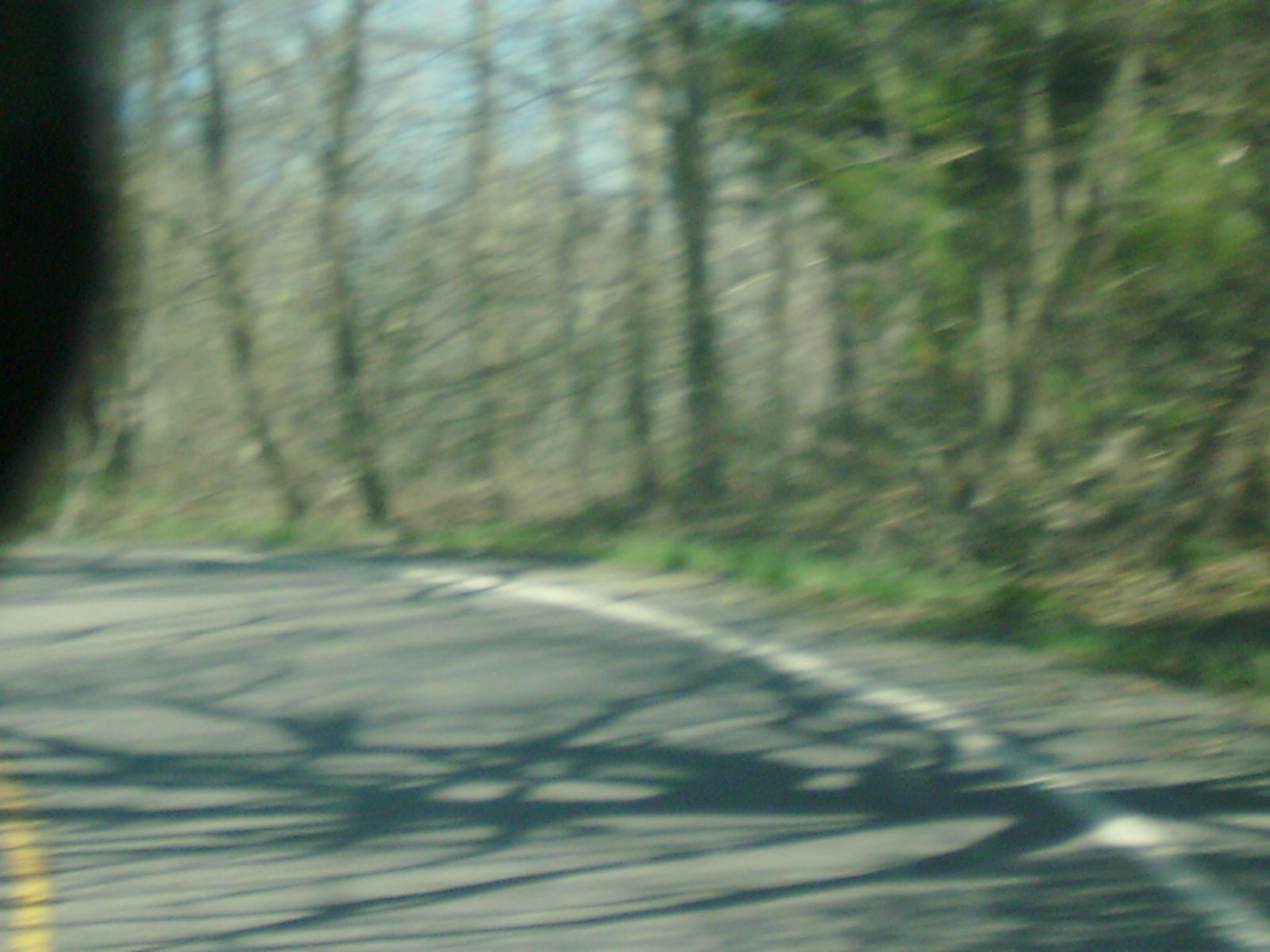This outdoor image, taken from the perspective of a driver on the right side of an asphalt road, captures the entrance to a curving roadway. The lower left corner reveals a faded yellow line, indicating a no-passing zone, while a solid white line starts in the lower right corner, curving leftward and exiting midway up the image, aligning with the road's bend. The setting is bright and sunny, casting clear shadows of tree trunks across the scene. The right side of the image displays a mix of greenery, with a bank of lush, evergreen trees amidst mostly bare deciduous trees, some of which have dried leaves. Sparse grass appears along the right shoulder of the road, with the terrain opening up halfway through the picture. The background features a hazy blue and white sky visible between the skinny brown branches of the mostly leafless forest. A dark shadow occupies the upper left corner, potentially obscuring part of the view, while the overall image remains slightly out of focus, enhancing the natural blur of a dynamic driving scene.